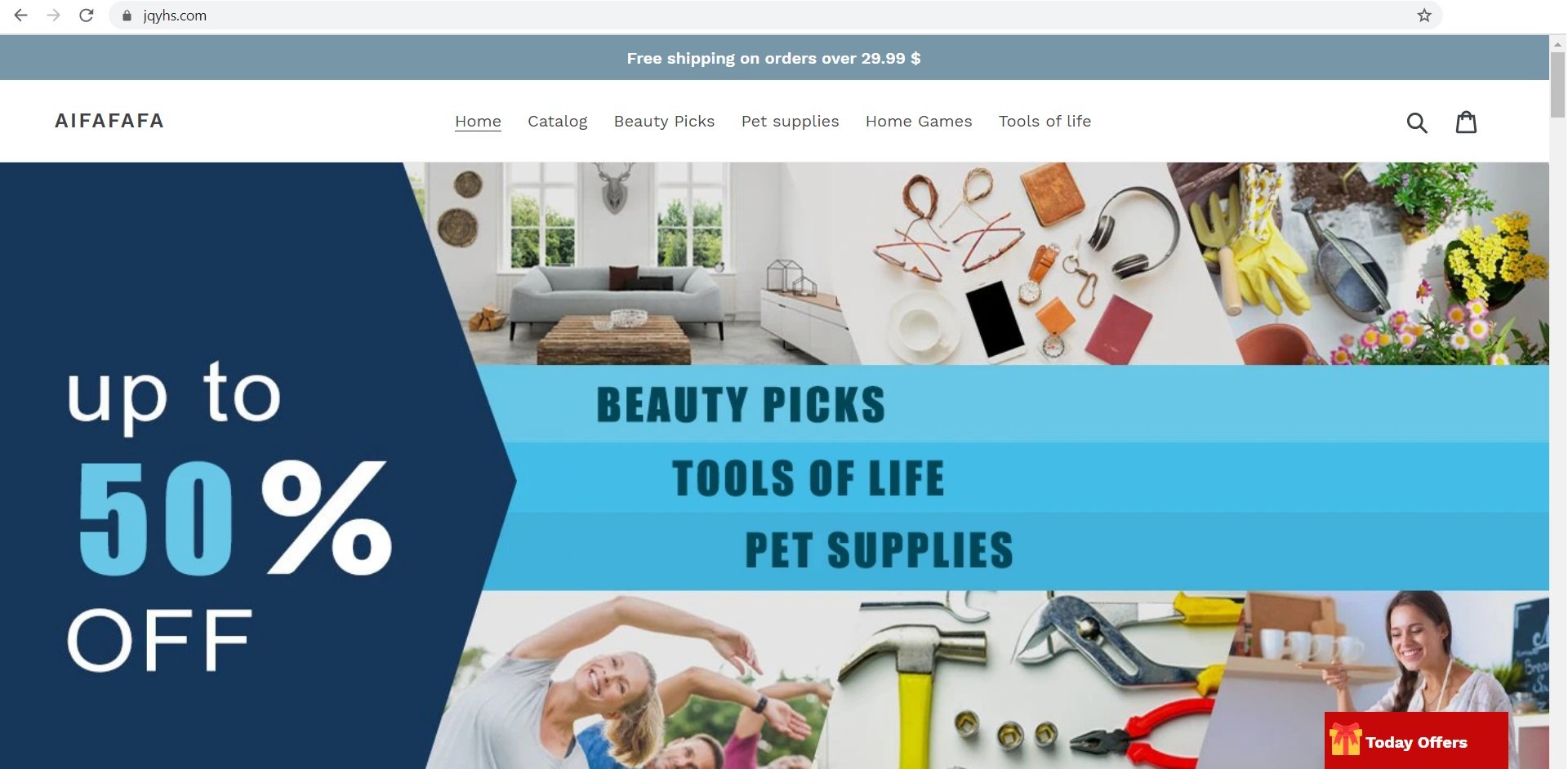Screenshot of an e-commerce website displayed on a desktop or laptop computer. At the top left of the screen, there are three icons: a gray arrow pointing to the left, a lighter gray arrow pointing to the right, and a gray refresh button. To the right of these icons, a horizontal, gray rounded oval spans about 90% of the horizontal space, featuring a gray outlined star.

Beneath the navigation bar, there's a grayish-blue rectangle with a promotional message: "Free shipping on orders over $29.99" in white text. Below this promotion, in all-capital blue letters, is the text "AIFAFAFA."

The website's main navigation menu includes several tabs: Home, Catalog, Beauty Pics, Pet Supplies, Home Games, Tools of Life, and Gray Text. The "Home" tab is currently selected, highlighted with a gray horizontal line underneath it. To the right of the menu, there is a darker gray magnifying glass icon and a dark gray shopping bag icon.

Prominently displayed to the right is a large blue pentagon, rotated so its point faces right, with the promotional text "Up to 50% off." The words "up to" and "off" are in white, while the number "50" is light blue.

The main content area includes six images in two rows, each showcasing different household items. Descriptions above these images are in dark blue text, categorized as "Beauty Pics," "Tools of Life," and "Pet Supplies," each set against a light blue rectangular background.